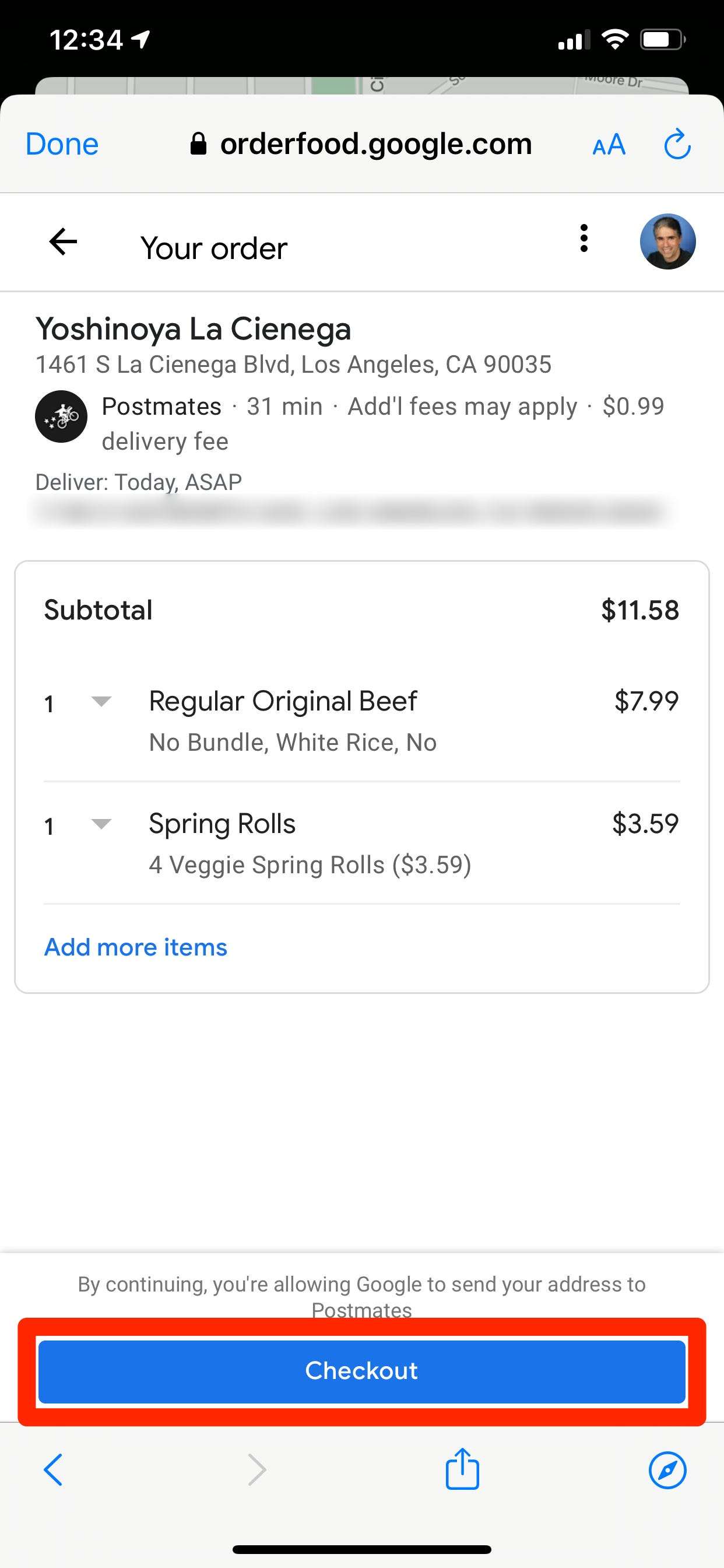Here is the cleaned-up and detailed caption:

---

A screenshot taken from the Safari browser on iOS shows a food order receipt from the Postmates delivery service. At the top of the screenshot, the current time is displayed as 12:34 on the left, accompanied by a location services icon, indicating that the device's location services are active. On the right side, there are icons for Wi-Fi or data connection and battery level. The main content of the screenshot reveals an order placed via the Google Maps interface, as indicated by the "orderfood.google.com" label. The interface includes clickable buttons labeled "Done," "AA," and a refresh button in blue.

The header reads "Your order," with a back arrow to return to the user's Google profile, a settings menu denoted by three vertical dots, and the user's profile icon on the right. The order is from Yoshinoya La Cienega, located at 1461 South La Cienega Boulevard, Los Angeles, California, 90035. Postmates estimates a 31-minute delivery time, subject to additional fees, with a base delivery fee of $0.99. 

The order details include a subtotal of $11.58, which comprises a Regular Original Beef with white rice priced at $7.99 and four veggie spring rolls costing $3.59. An option to add more items to the order is available. At the bottom of the page, there's gray text stating, "By continuing, you allow Google to send your address to Postmates," alongside a highlighted blue "Checkout" button outlined in red, indicating the action required to complete the purchase.